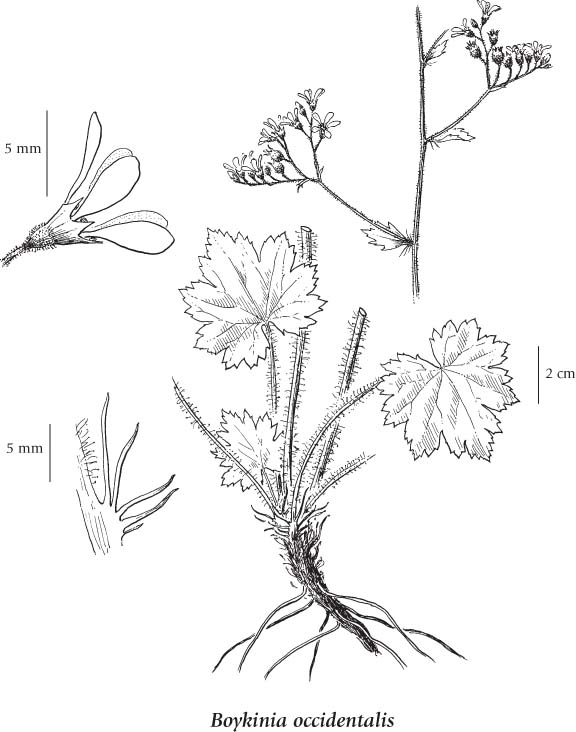The illustration is a detailed botanical sketch of *Boykinia occidentalis*, featuring multiple views and measurements. In the upper right corner, the main plant is depicted in black and white, with a central stalk branching into three segments, each bearing small flowers. To the left of this plant, there is an enlarged close-up of one of the flowers, accompanied by a scale bar indicating five millimeters. The lower right corner showcases another plant with a distinct root system; its stalk splits into several smaller stalks, three of which have leaves. Additionally, the image on the lower left includes a close-up of a segment showing the division of the stalk, marked with a five-millimeter scale. The diagram also highlights leaf details, resembling maple leaves, each approximately two centimeters wide. Overall, the illustration captures various aspects of the plant with precise botanical detail, emphasizing both the flowers and leaf structure.